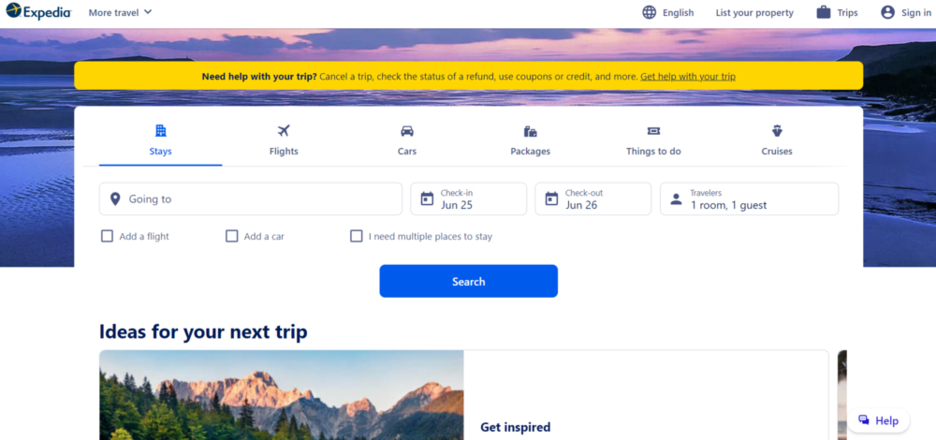The image depicts a webpage from the popular travel booking site, Expedia. The user has navigated to the "Stays" tab, indicating they are in the process of booking accommodation for a vacation. The primary section of the page offers various assistance options, including cancelling a trip, checking the status of a refund, using coupons or credits, and more.

Currently, the booking section displays preliminary details: one room for one guest, with dates specified from June 25th to June 26th. However, the location field remains unfilled, prompting the user to input additional information before proceeding with the search for available rooms. Directly beneath the search button is a section labeled "Ideas for your next trip," which suggests various popular tourist destinations for potential travelers.

The page also highlights the breadth of services Expedia offers: users can book not only accommodations but also flights, car rentals, vacation packages, activities, and even cruises. This comprehensive platform provides all the necessary tools to plan an entire trip in one place.